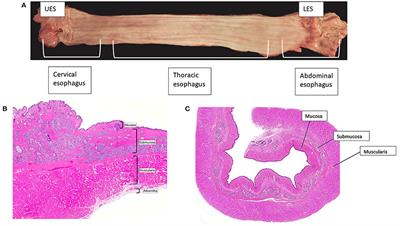The image is a detailed anatomical chart of the esophagus, set against a black background. At the top of the image, initials "UES" (Upper Esophageal Sphincter) and "LES" (Lower Esophageal Sphincter) are indicated. Below these, the esophagus is divided into three labeled sections: cervical esophagus, thoracic esophagus, and abdominal esophagus. 

Below this main diagram, there are two smaller images labeled "B" and "C":

- Image B, on the left, shows a pink representation, whose details are too small to read.

- Image C, on the right, also shows a pink representation, featuring several white boxes with black writing pointing to specific areas, presumably indicating different anatomical features or tissue types of the esophagus.

The chart seems to provide a comprehensive look at both the overall structure and cross-sectional details of the esophageal tissue, showcasing the various components from the outer layers to the innermost parts.